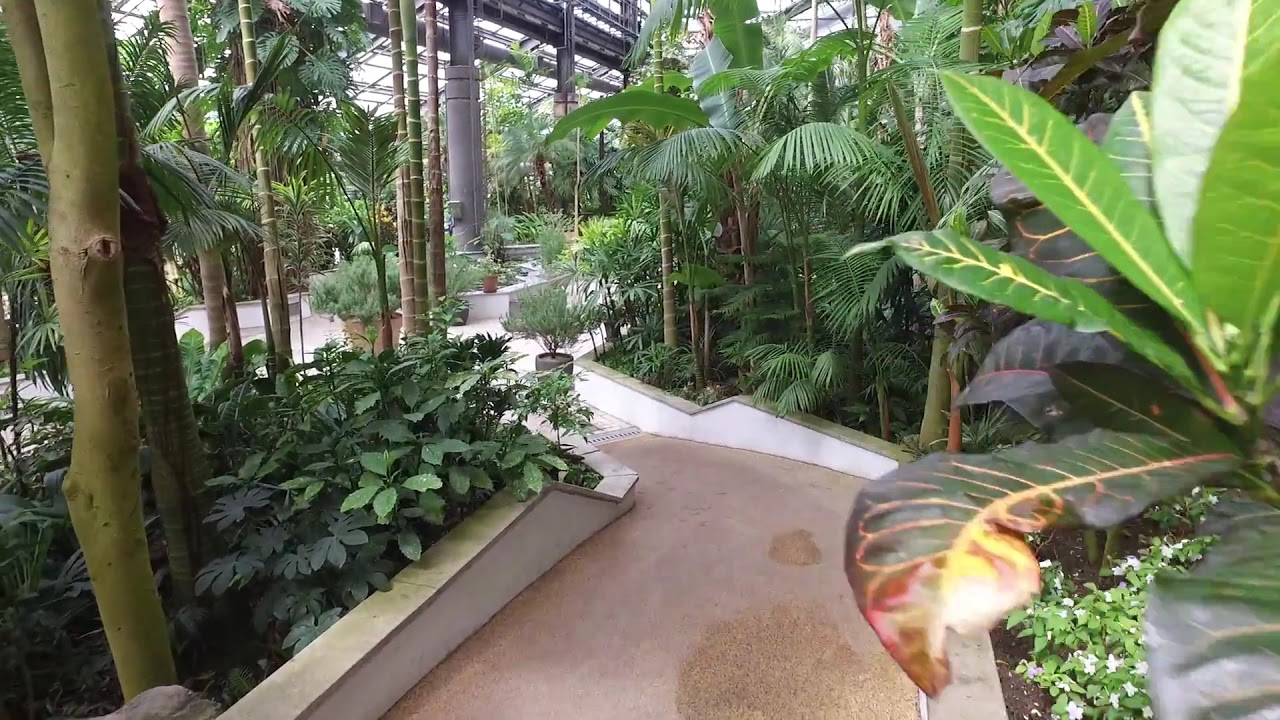This image captures the vibrant interior of a large greenhouse or botanical pavilion, characterized by a variety of lush tropical and fern trees, as well as numerous other plant species. The indoor setting is evidenced by the transparent roof and walls, through which natural light floods the space, ideal for sustaining the dense greenery. A pathway, slightly pinkish-red in hue with white railings topped by brown surfaces, winds through the foliage, leading the viewer's eye around the display of verdant plants. Alongside the path, there are tropical trees featuring palm fronds and leaves of various greens and reds, their trunks standing tall amidst the dense undergrowth. At the center, a small pond adorned with a flower pot possibly contains lily pads and fish, adding to the serene ambiance. The scene is devoid of people, emphasizing the tranquil, almost untouched natural beauty within this carefully curated indoor garden. There are even steel beams or struts at the top, part of the greenhouse structure, providing support and adding to the industrial charm of this verdant oasis.